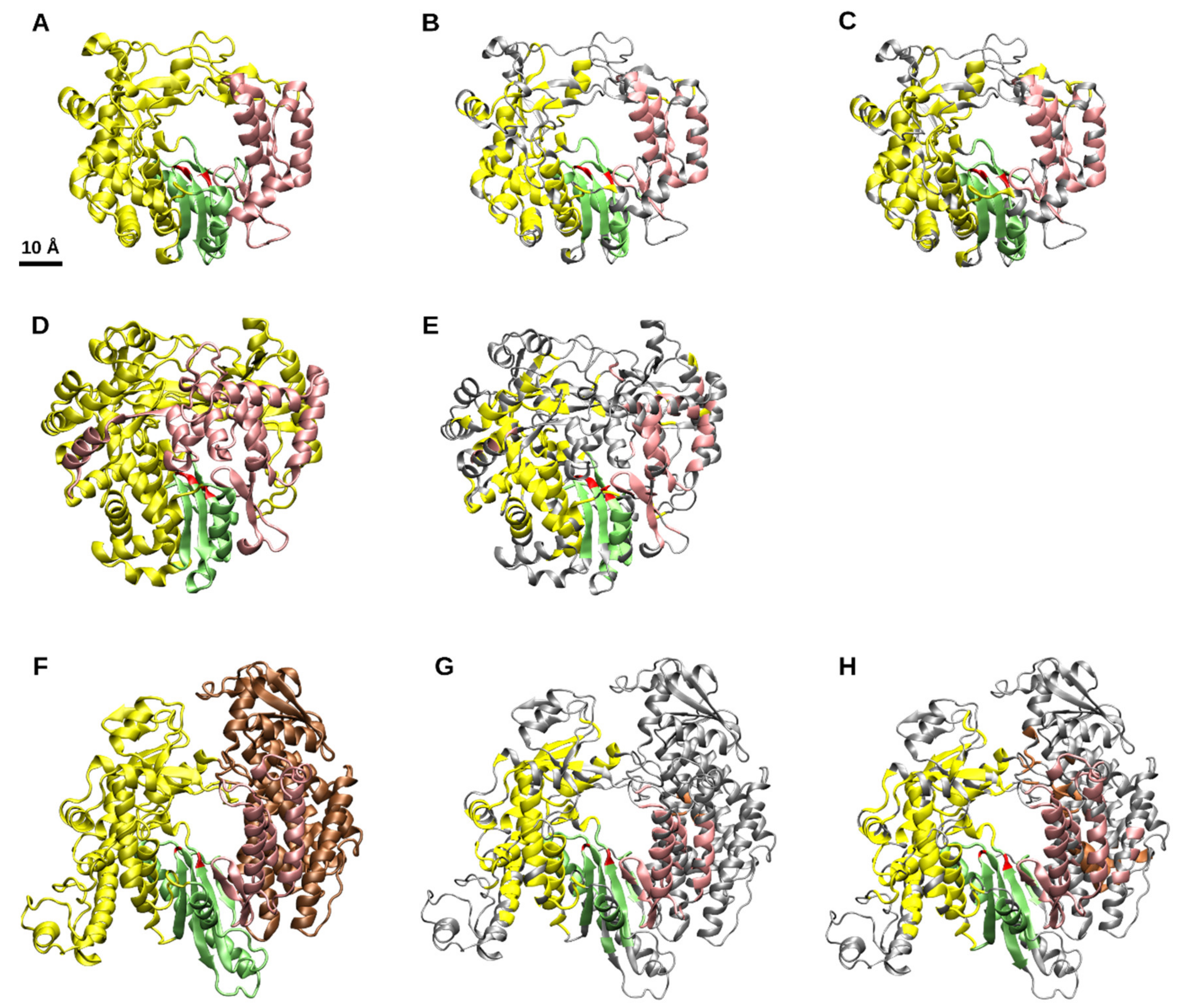The image depicts a well-organized series of vibrant, curly decorations, which resemble crumpled and colorful ribbons or garlands. These decorations are arranged in a structured diagram format and labeled with letters from A to H. The first row contains items labeled A, B, and C; the second row contains D and E; and the third row contains F, G, and H. 

Each decorative item showcases a blend of yellow, green, and pink colors, with some variations like a brown shade on the bottom row. The items appear to increase in size and complexity from top to bottom. The decorations in the top row are relatively simple and circular, while those in the bottom row (F, G, H) are larger, with some looking more detailed and intricate, possibly resembling small animal shapes crafted from the ribbon-like material.